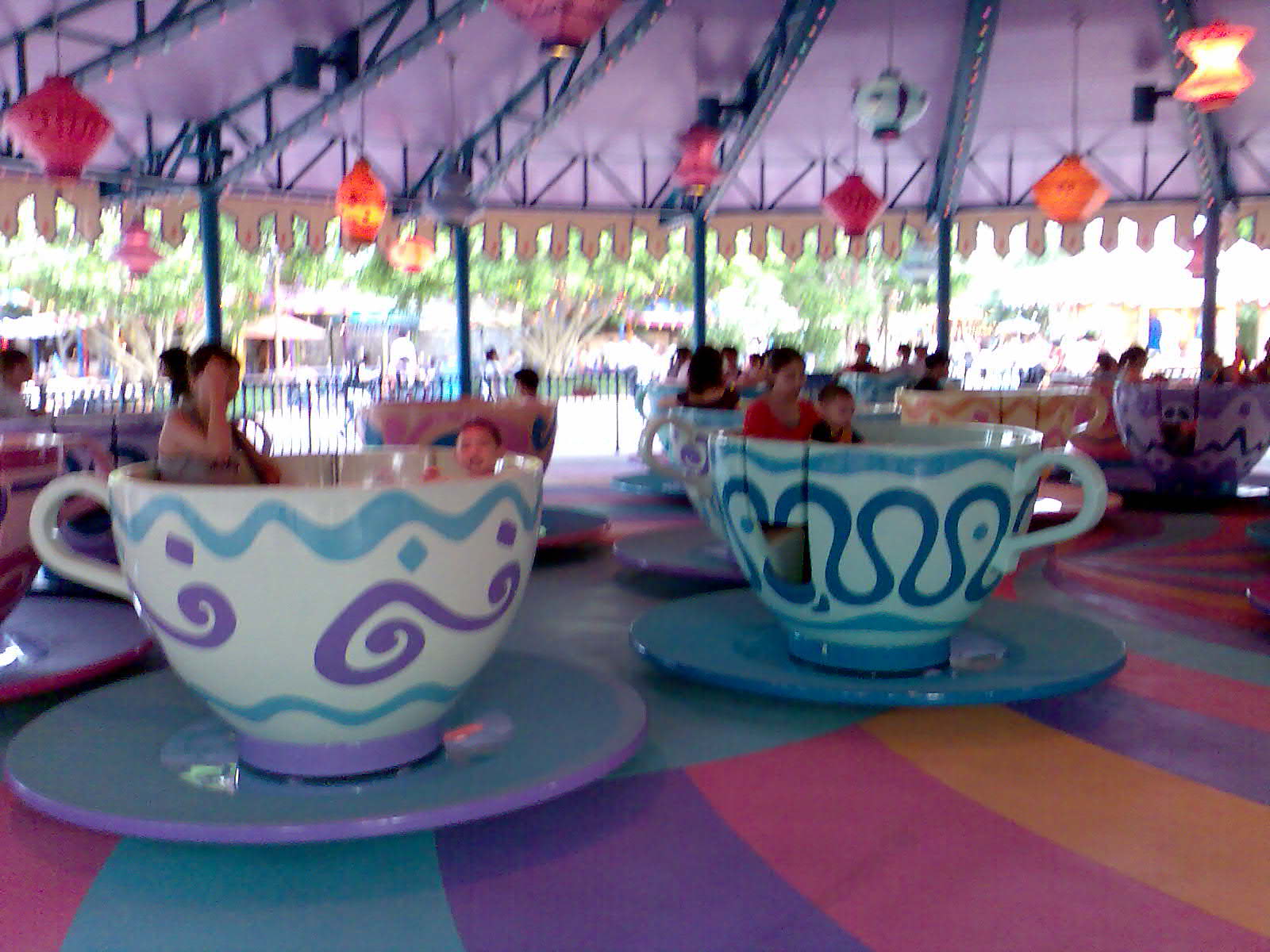This vibrant photograph captures a whimsical teacup ride at an amusement park, set under a light purple fabric awning adorned with colorful Chinese-style paper lanterns. The ride features large, white teacups embellished with blue and purple designs, each perched on equally oversized saucers, positioned on a brightly striped floor showcasing shades of blue, aqua, fuchsia, and orange. The teacups, seen in motion, create a slight blur in the image, enhancing the sense of dynamism and fun. Inside the teacups, various individuals—mostly parents with children, all in summer attire such as tank tops and t-shirts—enjoy their ride. Beyond the charming, enclosed ride area, the outdoor scene reveals green trees, carnival booths, and vendors with umbrellas, further emphasizing the festive atmosphere of the amusement park.